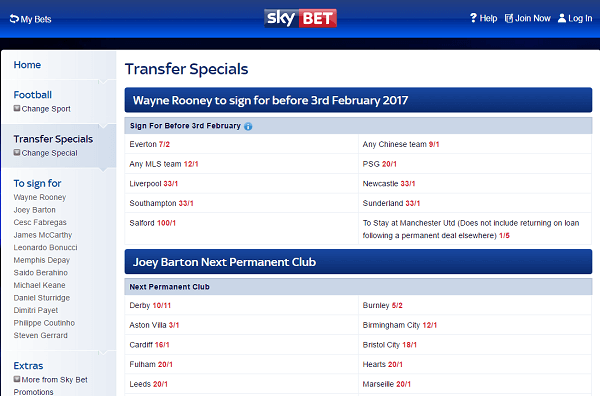The webpage features a clean design with a white background. At the top, a blue banner spans across the page. On the left side of this banner, it displays the text "MyBats" while the center reads "SkyBats". On the right side, there is a question mark icon accompanied by the word "Help". Next to this, a square icon with a pencil inside indicates the "Join Now" option. Further right, a people icon is paired with the text "Log In".

Below the banner, the left-hand side of the page features a vertical menu with blue tabs. The tabs are labeled as follows:
- **Home**
- **Football**
  - Under the "Football" tab in black text, it says "Change Sport"
- **Transfer Specials** (highlighted as the selected tab)
- **To Sign For**
- **Extra**

The main content of the page is dedicated to "Transfer Specials". It includes a section with a blue rectangle containing white text that reads: "Wayne Rooney to sign for before 3rd February 2017". Below this, a list of possible teams is provided: Everton, any MLS team, Liverpool, Southampton, Saffron. Another section beneath this, also within a blue rectangle, is titled "Joey Barton next permanent club".